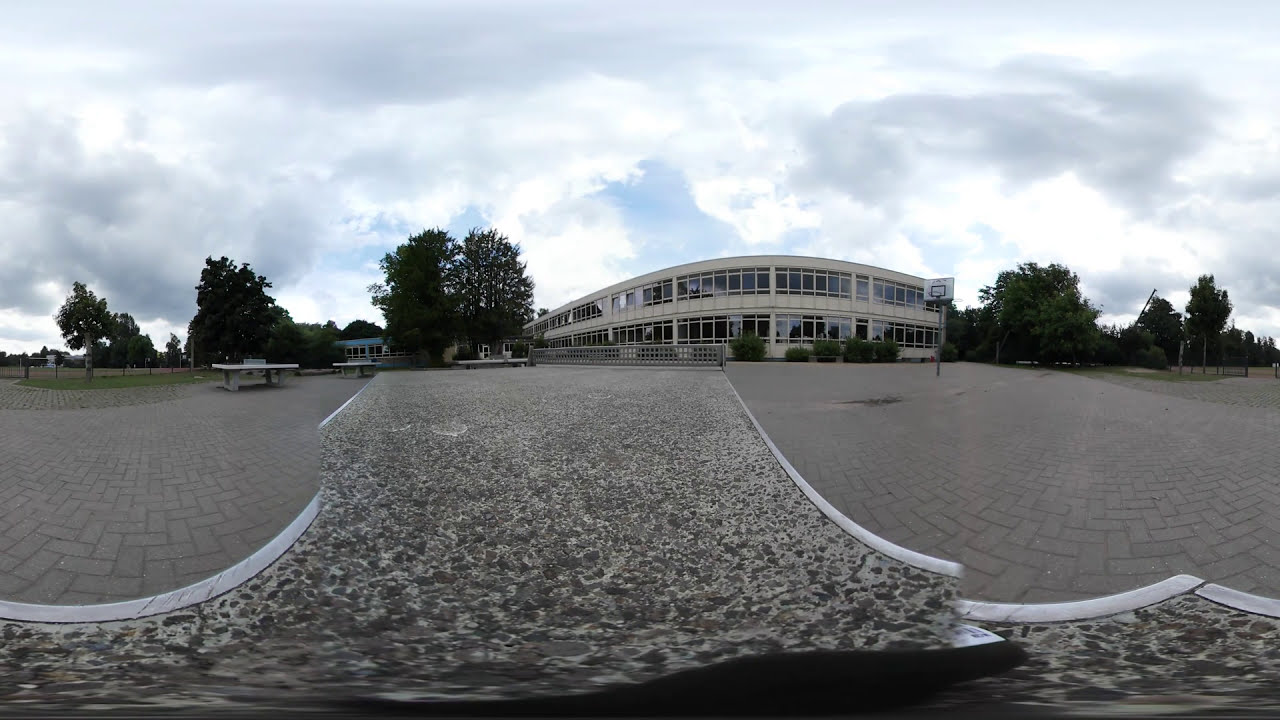The image showcases a panoramic view of a large commercial courtyard area in front of an extensive two-story building that spans the entire width of the picture, although part of it is cut off. The building has a distinctive modern design with numerous windows on both floors and sections painted blue. Directly in front of the building lies a vast gray and brown cobblestone walkway, outlined with brick gray pavers, leading into a consolidated gravel path that blends seamlessly with the courtyard's surface. 

Dominating the right side of the composition, there is an old basketball hoop positioned on a metal pole with a white backboard. Stone tables and several benches are scattered throughout the area, with three benches specifically noted off to the left side, adjacent to a grassy patch. In the distance, sparsely planted tall green trees frame both sides of the courtyard, adding a touch of nature to the scene. The sky above is predominantly blue, punctuated with thick, white, and light gray clouds, suggesting an overcast day with the sun attempting to break through.